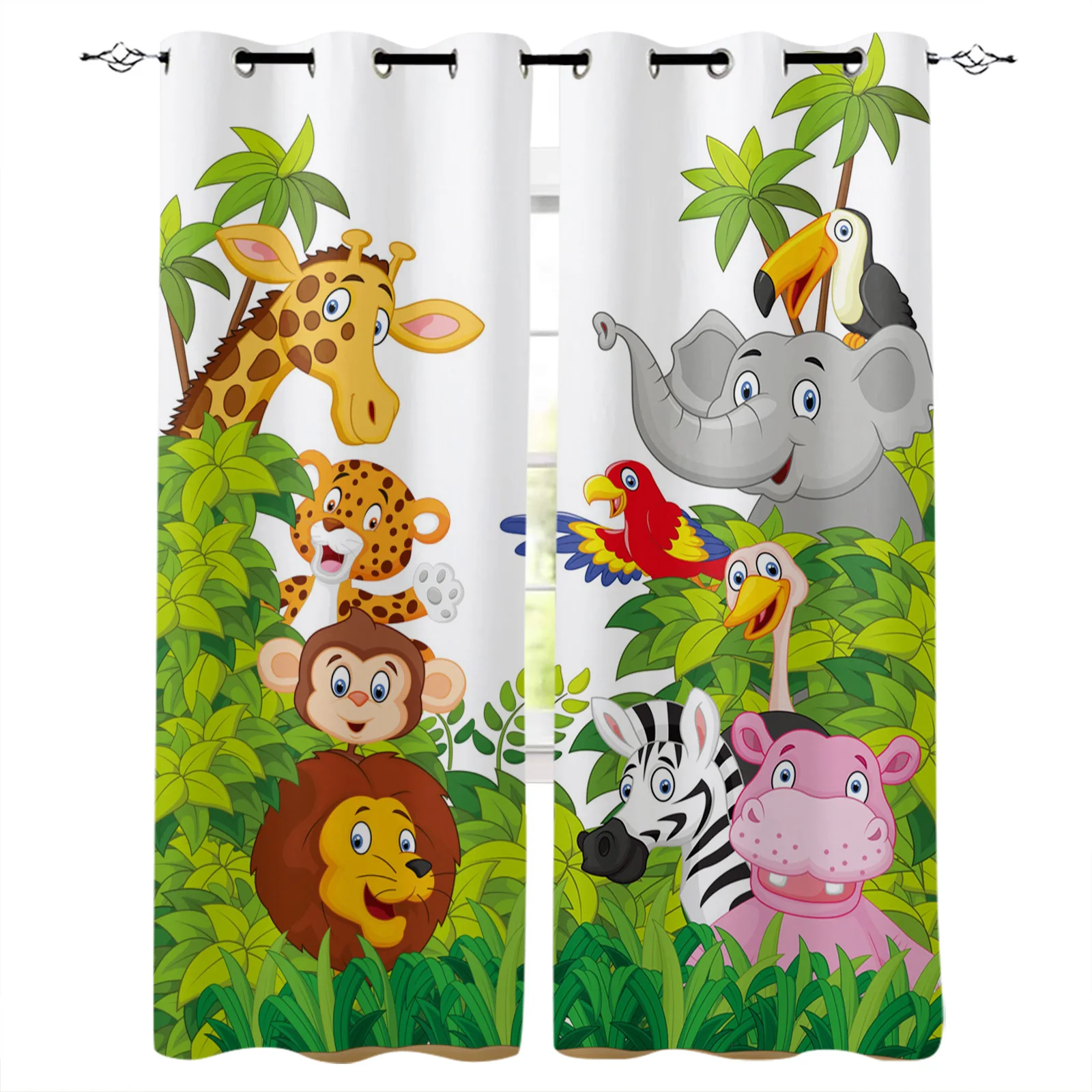This image features a vividly colored children's style curtain, ideal for a product listing on a retail website. Suspended from a sleek black metal curtain rod using silver grommets, the curtain comprises two panels adorned with whimsical cartoon jungle animals against a bright white background. 

On the left panel, from top to bottom, the design includes a cheerful yellow giraffe, a friendly waving cheetah cub, a playful monkey with large ears, and the head of a peeking lion surrounded by lush green leaves and grass. 

The right panel showcases more delightful creatures: a toucan perched atop a gray elephant, a vibrantly feathered parrot in red, yellow, and blue, a curious ostrich, and at the bottom, a zebra with classic black and white stripes standing next to a pink hippopotamus. The scene is framed by abundant green foliage, adding to the jungle theme and creating an engaging, playful atmosphere perfect for a child's room.